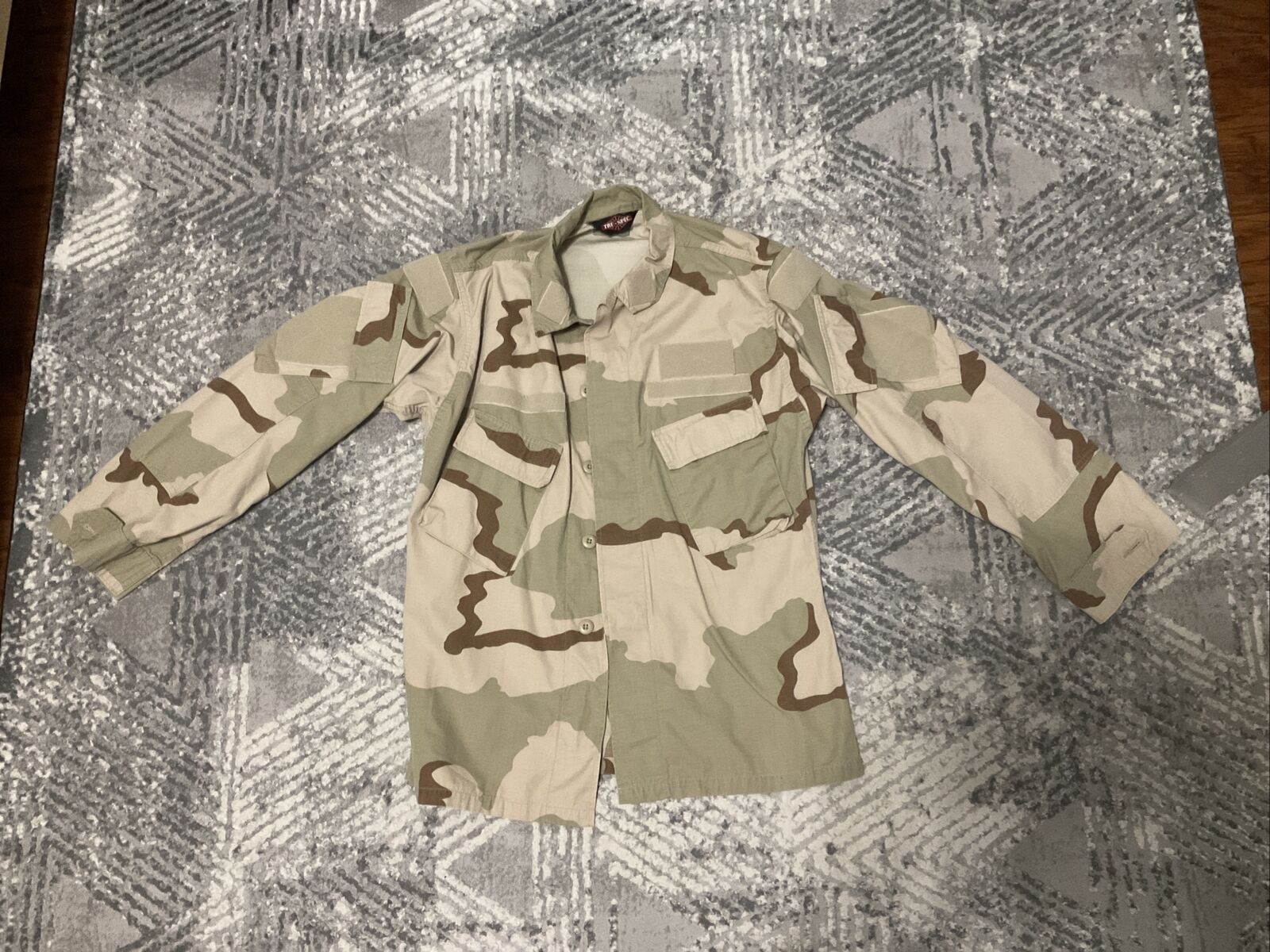The photograph features a long-sleeve, military-style camouflage jacket laid out flat on a surface covered by a patterned throw rug. The jacket, which has a collar and unfastened tan buttons down the front, is designed with a desert camouflage pattern comprising wavy blobs in olive green, light tan, and chocolate brown. The surface beneath the jacket is a gray throw rug adorned with an X-pattern composed of various shades of gray and white, giving it a textured and intricate appearance. Small portions of the wooden floor are visible on either side of the rug, framing the scene. The jacket is positioned on its back with the sleeves spread out to the sides, and no identifiable military insignia or emblems are present on the garment.